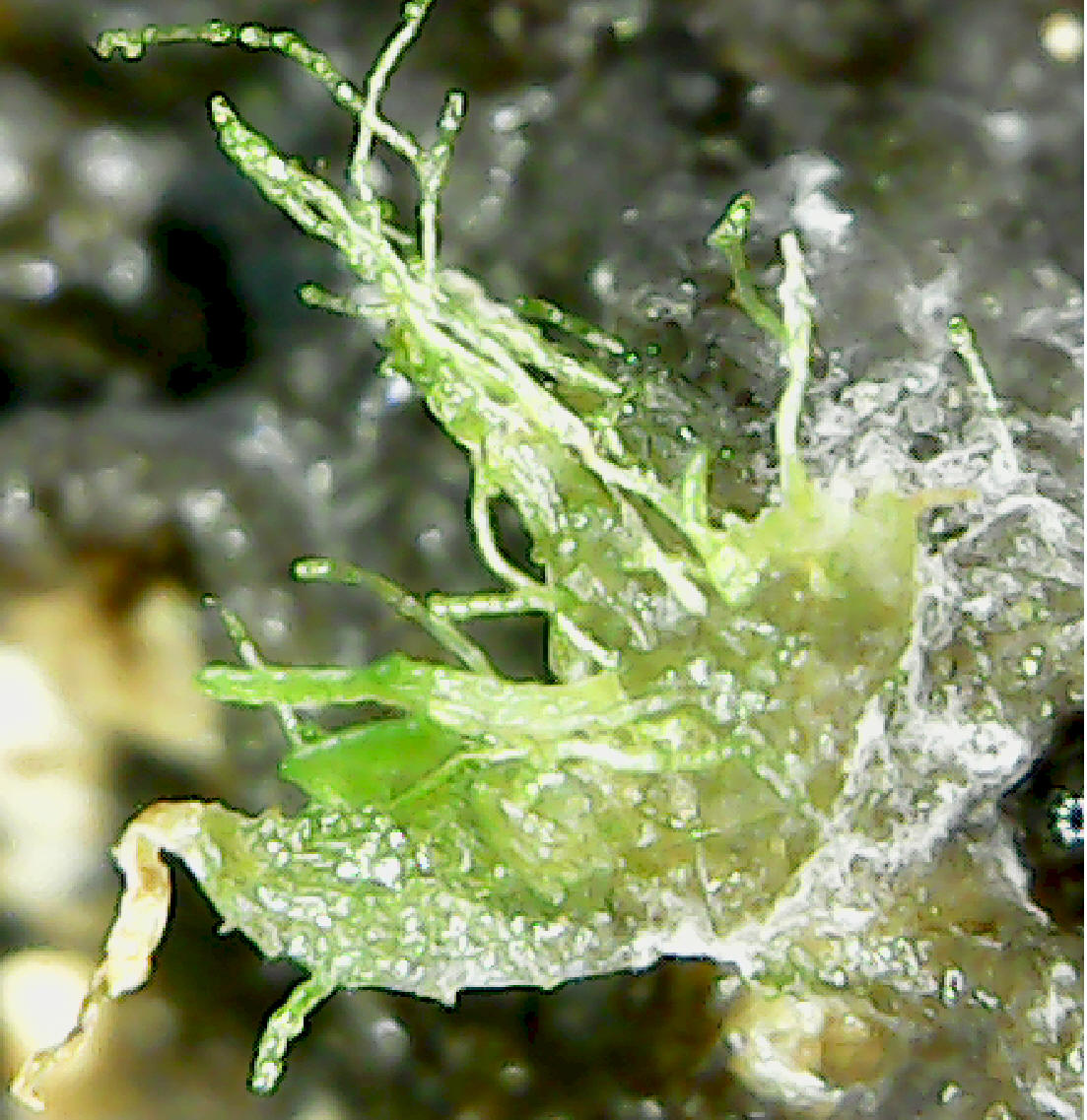A dynamic, gritty, and out-of-focus color photograph captures a burst of water splashing upward and outward from a green object, possibly a lime slice. The water gushes forward in vibrant green and yellowish tendrils, interspersed with flecks of white foam that add a sense of movement and energy. These foamy flecks continue into the blurred background, which features a darker shade of green and accentuates the lighter, detailed splashes in the foreground. The chaotic yet mesmerizing scene suggests a lime being squeezed, with juice spraying in all directions. In the lower left side of the image, light filters in, adding depth and highlighting the dynamic spray pattern of the liquid.